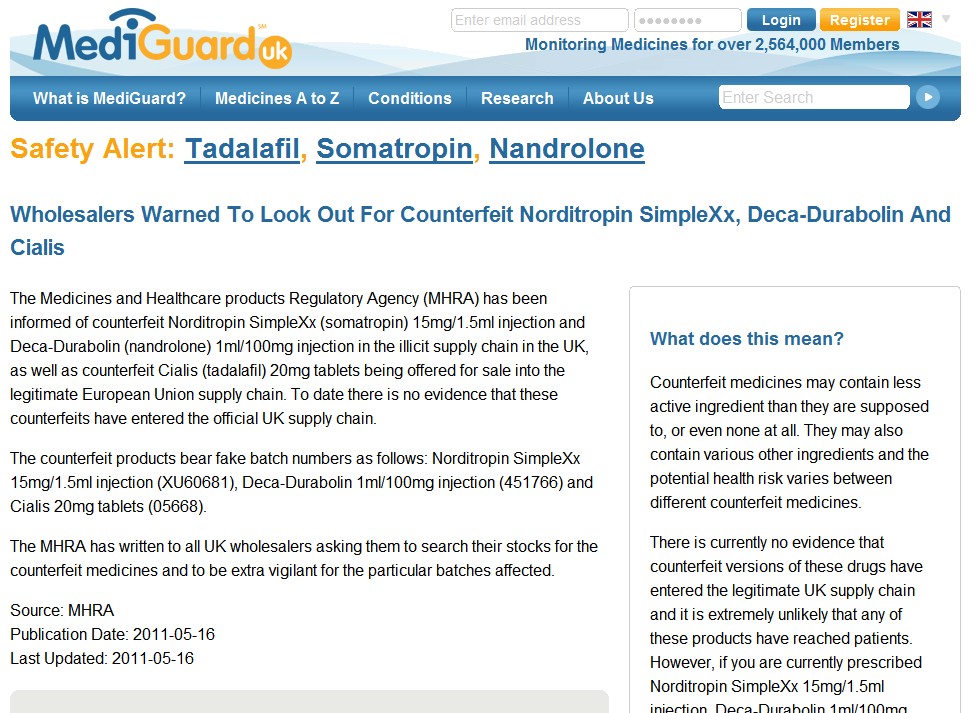Below is the refined and detailed caption for the described image:

---

The image is a detailed screenshot of the MediGuard UK webpage. At the top left corner, the logo "MediGuard" is prominently displayed, with "MEDI" in blue and "Guard" in orange, separated by a blue arch over the letter "I". Adjacent to this logo, there is a small, orange circle containing the letters "UK" in white text.

The top section of the webpage features login credentials fields—an input box labeled "Enter email address" followed by another for "password". To the right of these fields are two buttons: a blue "Login" button and an orange "Register" button, alongside the UK flag icon.

Beneath these options, in blue text, is a statement indicating the platform's reach: "Monitoring medicines for over 2,564,000 members." Below this statement runs a horizontal blue navigation bar with several tabs: "What is MediGuard," "Medicines A-Z," "Conditions," "Research," and "About Us". On the far right of this bar is a search box labeled "Enter search."

Directly under the navigation bar, the term "Safety Alert" appears in bold, orange text. Following this is a list of three medications—Tadalafil, Somatropin, and Nandrolone—each underlined and separated by orange commas. 

A subhead in blue text states: "Wholesalers warned to look out for counterfeit Nordotropin SimpleXX, Decadurabolin, and Cialis." The notification informs that the Medicines and Healthcare Products Regulatory Agency (MHRA) has detected counterfeit versions of Nordotropin SimpleXX Somatropin 5MG/1.5 ML injection, Decadurabolin Nandrolone 1ML 100MG injection, and Cialis 20MG tablets within the illicit supply chain in the UK. However, it clarifies that there is currently no evidence suggesting these counterfeit medicines have infiltrated the official UK supply chain or the legitimate European Union supply chain.

---

This caption provides a comprehensive overview of the webpage contents and their layout.